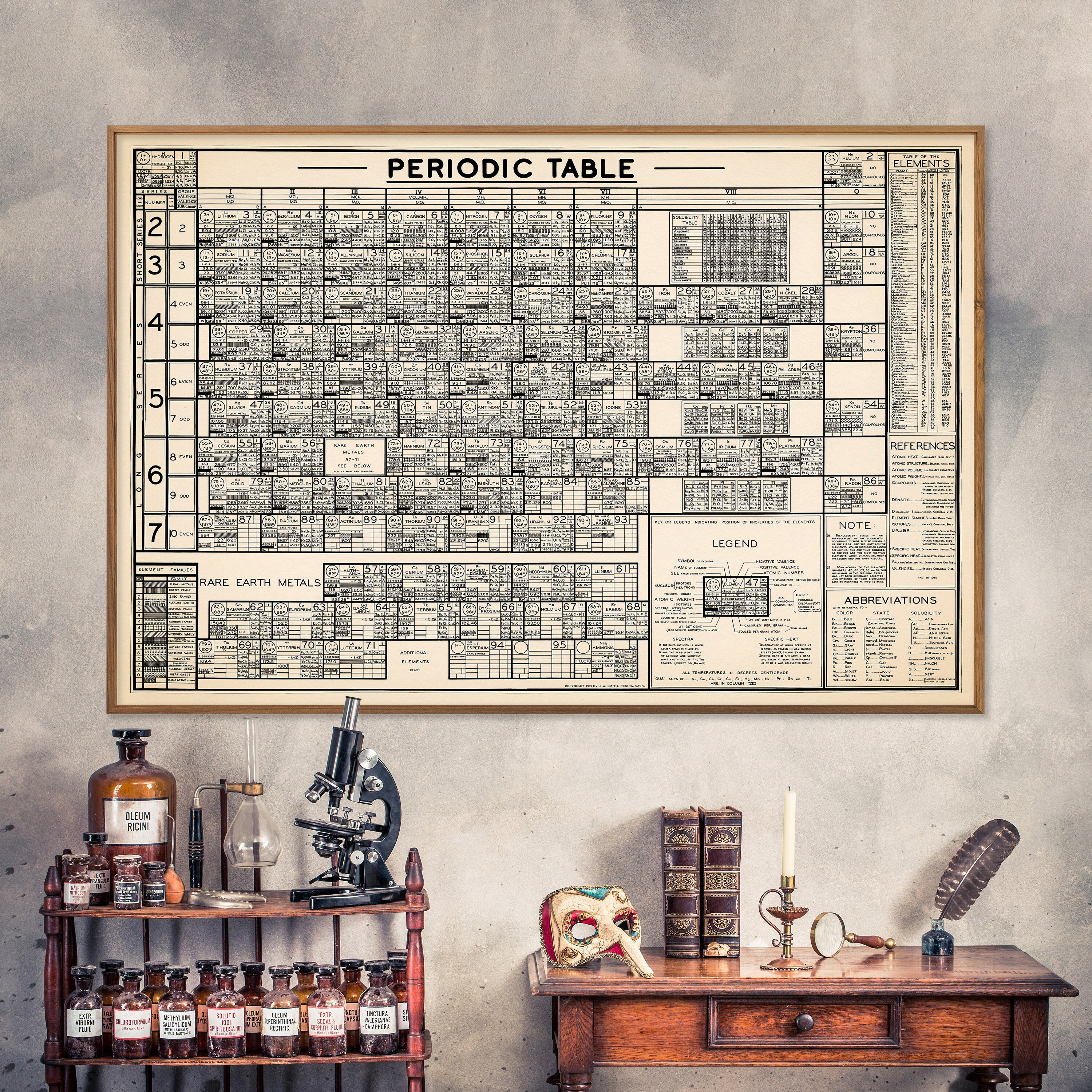The image depicts an intricately detailed, vintage-style chemistry lab. The background consists of a gray marble-textured wall, occupying the upper two-thirds of which is a wooden-framed, antique-looking poster of the periodic table. The table, labeled "Periodic Table" in black, old-style text, comprises various rows numbered 2 through 7, and includes a section detailing rare earth metals along with a legend on reading the table and a note on abbreviations.

At the bottom left of the image is a wooden shelving unit adorned with numerous labeled bottles. The most prominent among them is a large brown bottle labeled "Oleum Racini." The shelf also hosts a black microscope and a beaker apparatus. To the right, there is an antique wooden dresser. Items on the dresser include a white Venetian-style mask with a long curved beak, two upright tomes, a bronze candlestick holding a white tapered candle, a magnifying glass, an inkwell with a quill pen, and an assortment of other vintage scientific instruments. The setting evokes a nostalgic, historic chemistry lab atmosphere, blending scientific tools with elements of classical elegance.